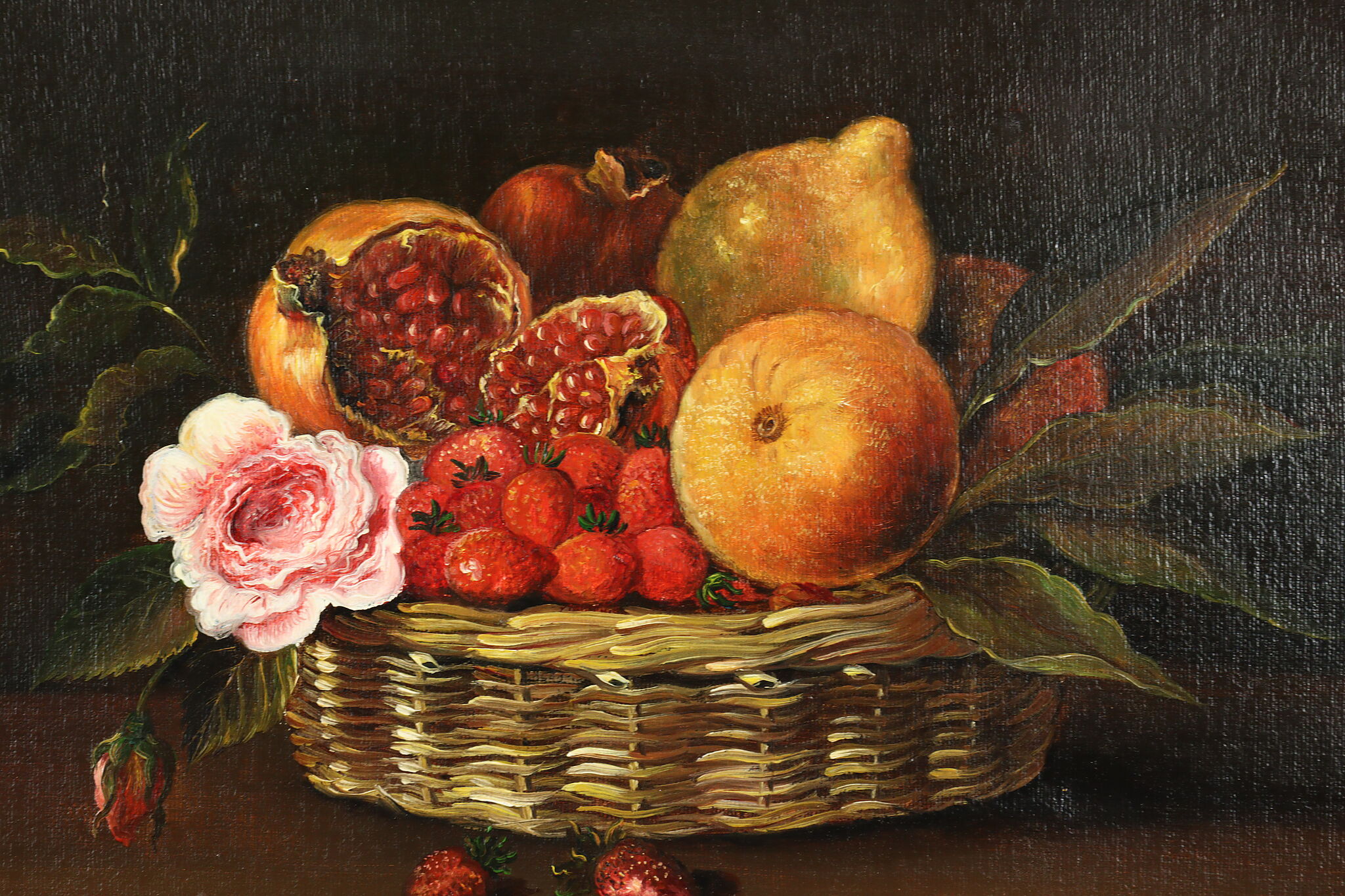This is an oil painting of a classic still life featuring a low-profile woven brown basket filled with an array of vibrant fruits and flowers, set against a dark background that transitions from black to deep brown at the bottom. The basket, centrally positioned, contains a rich assortment of items: a prominent pink flower and a wilting rose extend from the left, while a split pomegranate reveals its seeds on the top right. Behind the pomegranate, a tan persimmon and a partly visible lemon can be seen, with an orange nestled in front of them. Central within the basket is a cluster of bright red strawberries, some of which have fallen out onto the table below, adding a realistic touch to the composition. Dark and leafy green foliage protrudes from both sides of the basket, enhancing the depth and classical feel of the painting. In the back right corner, an indistinct orangey-red fruit adds a splash of color and intrigue. The overall composition, with its rich saturation and interplay of light and shadow, conjures the mastery reminiscent of old European still life paintings.